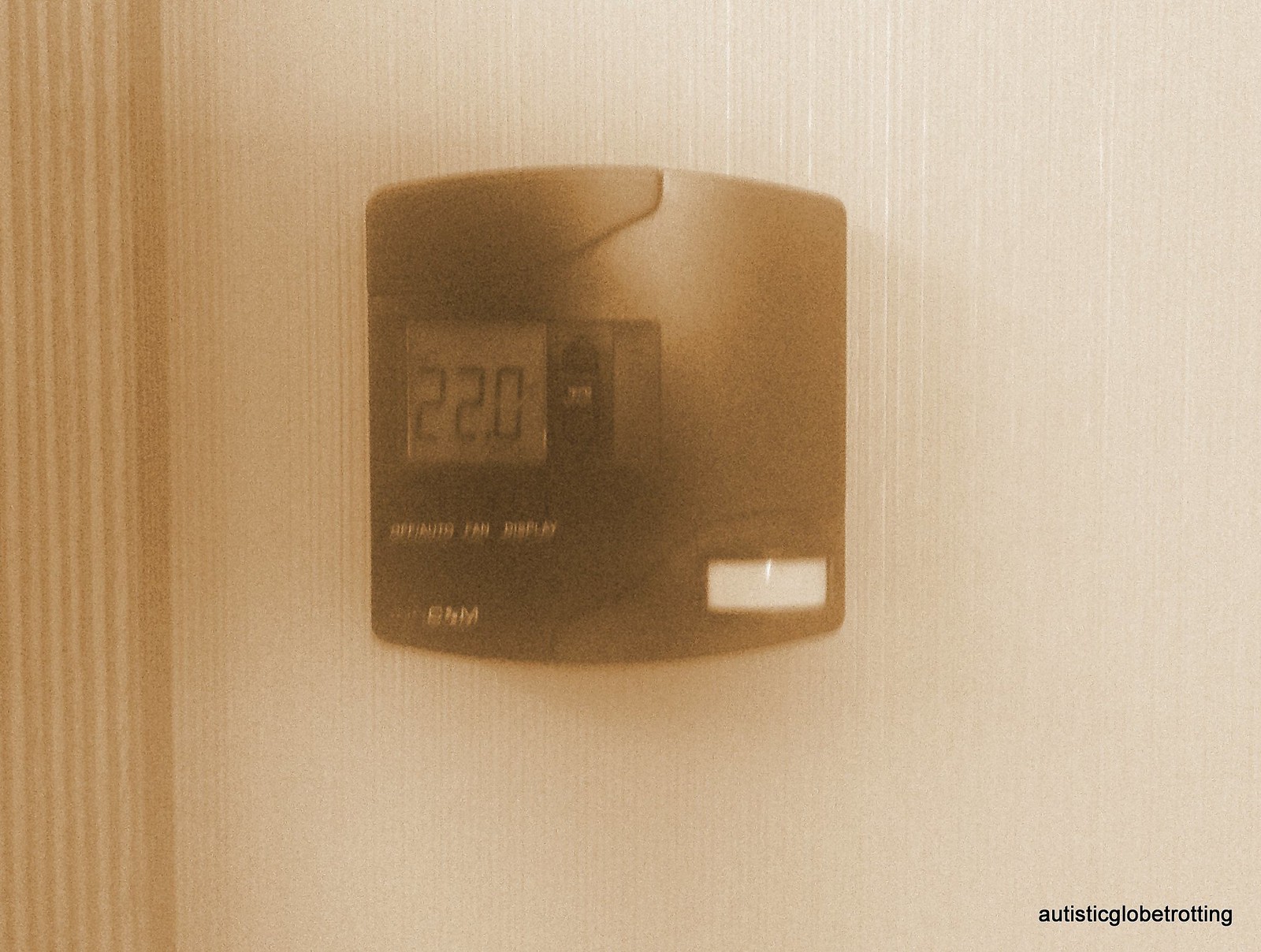The image features a rectangular photograph with a yellowish filter, presenting a square-shaped plastic thermostat centrally mounted on a textured gray wall. The photograph, along with the thermostat, appears blurry and out of focus. The thermostat displays multiple white words such as "off/auto", "fan", and "display", alongside an indistinct logo in the bottom left corner.

A gray LED screen on the left center of the thermostat reads "22.0" in black digital numbers. Adjacent to the screen are two rubber buttons featuring upward and downward arrows, likely for temperature adjustment. The bottom right corner of the thermostat includes a white plastic rectangle, probably serving as a motion sensor. Overlaying the bottom right corner of the photograph is black text reading "autistic globe trotting."